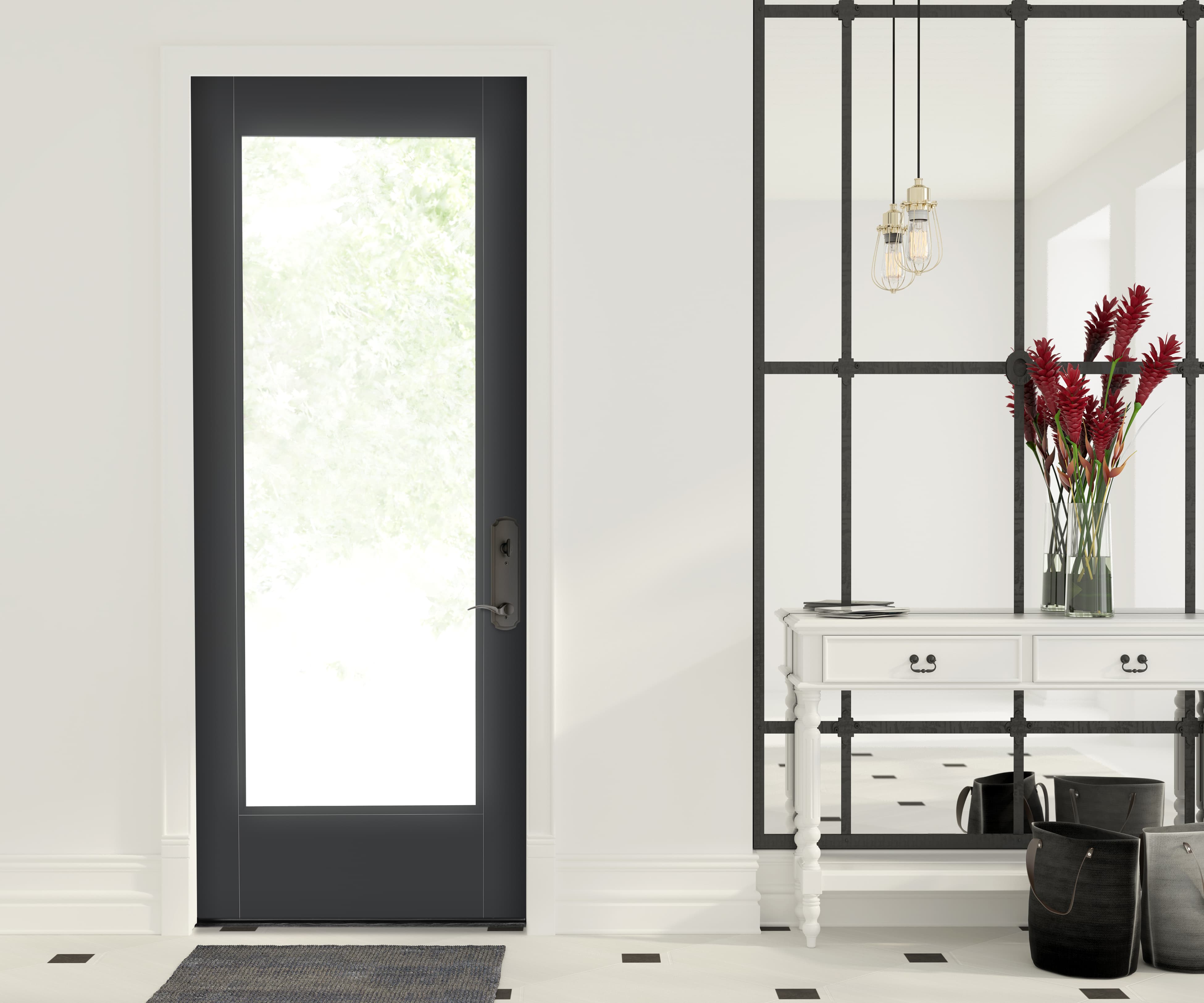The image showcases the interior of a house, focusing on a front entryway. On the left, there's a door with a large glass pane framed by a dark gray or black surround, complemented by a small gray doormat. Through the glass, a tree can be seen outside. The floor is predominantly white with a pattern of small black squares, suggesting it is tiled. The white wall provides a clean backdrop.

To the right of the door, there is a long, narrow entryway table with two drawers featuring black handles. The table is adorned with a clear vase holding red long-stemmed flowers. Behind the table stands a large mirror with a black crisscross design at the top, extending high, possibly out of the frame. Above the scene, two light fixtures with Edison bulbs hang down, adding a vintage touch.

On the floor in front of the table are two bags—one with straps, possibly a black tote, and another gray square object that could be a trash can. The setup is neatly arranged, combining modern and classic elements in the entryway décor.